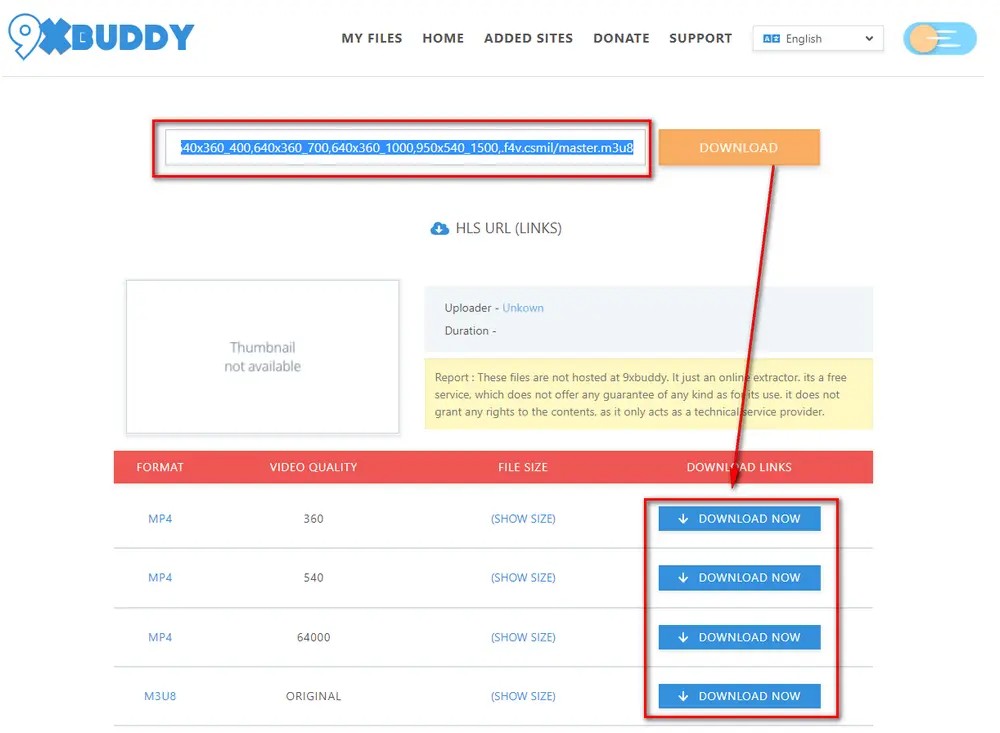The image captures a screenshot of the 9xbuddy website, a media download platform. At the top of the page, there is a navigation bar containing various links: "My Files", "Home", "Added Sites", "Donate", and "Support". To the right of these links, there is a language selection dropdown menu, with English currently selected. Below this menu, there is an input field where users can paste a link to download content.

The primary function of the website appears to be media downloading. Towards the bottom of the page, a table displays different video formats, quality options, and corresponding file sizes, with download links for each format. The screenshot also reveals that there is an area designated for displaying video thumbnails, but it currently shows "Thumbnail not available". Various sections of the website are highlighted to guide users on how to proceed with their downloads.